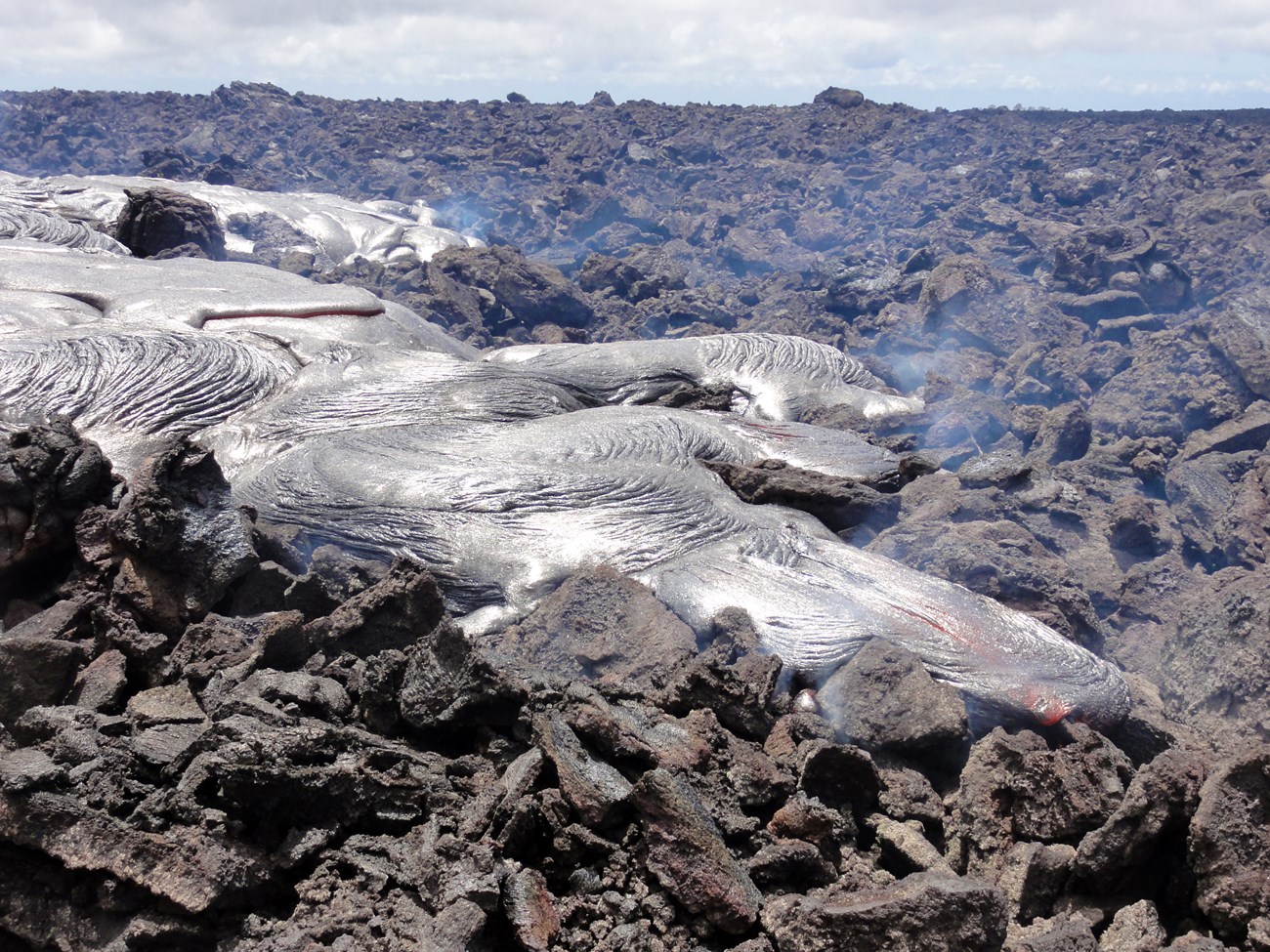In this detailed image, we see freshly erupted lava, primarily originating from the upper left corner and flowing diagonally towards the bottom right. The lava, initially a smooth, liquid, gray-black mass, bears stark swirls and ripples indicating its slow, relentless movement. Interspersed with hues of light gray and occasional hints of yellow-orange at the edges, the lava illustrates areas where it's still intensely hot. Smoke and steam rise from several points, particularly from the center and the right end, signifying active cooling. The foreground and surrounding areas are dominated by dark, jagged, and bumpy rocks, remnants of previous lava flows now solidified into various shapes and sizes. These hardened lava formations resemble a rugged, barren landscape. The background features a clear blue sky dotted with a few clouds, offering a contrasting backdrop to the dynamic, fiery spectacle in the forefront.